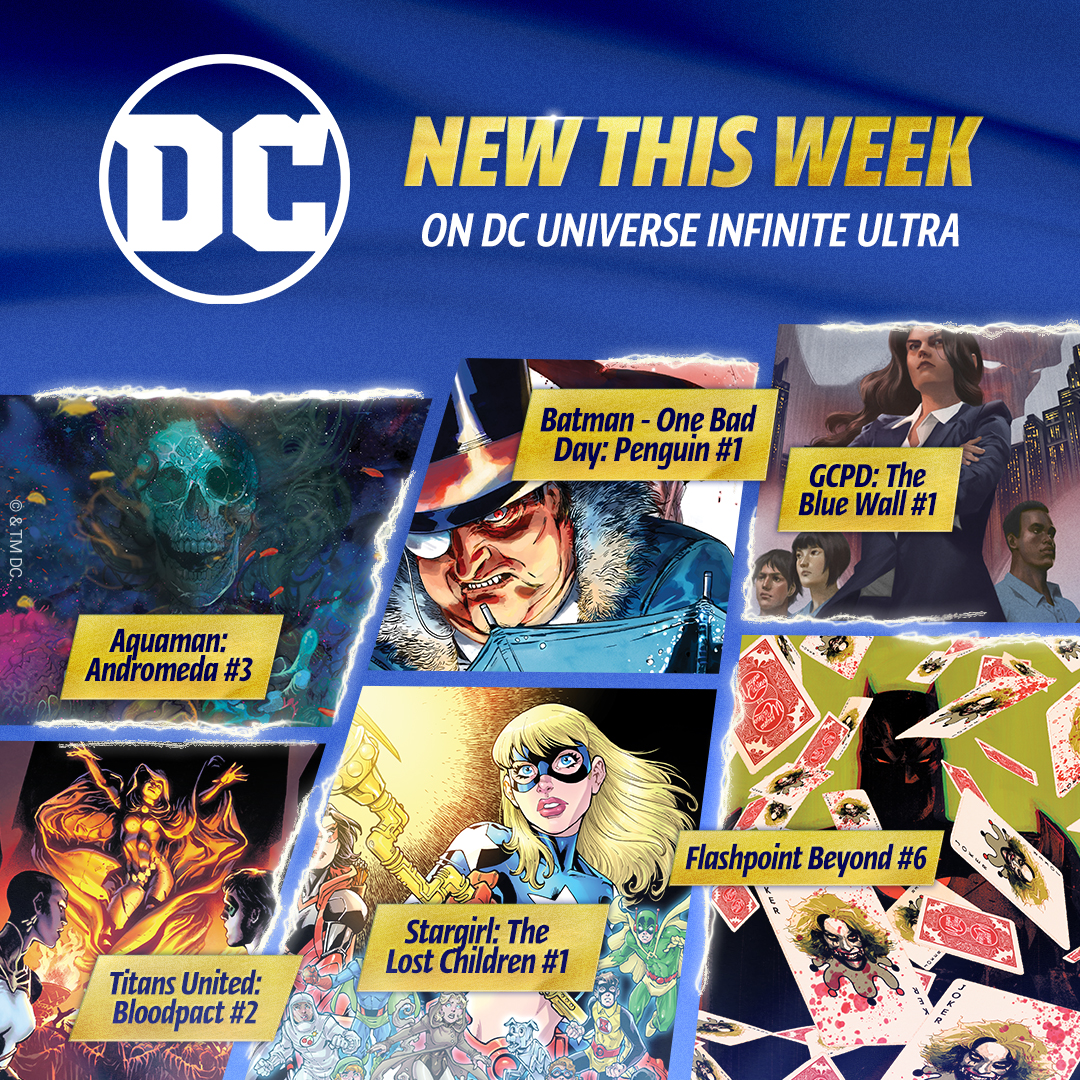The image is a collage-style advertisement poster for new comic releases on DC Universe Infinite Ultra, with the DC logo prominently displayed at the top. Below the logo, the header announces "New This Week on DC Universe Infinite Ultra" in a gold and white color scheme. The poster features six distinct panels, each highlighting a different comic issue:

1. Aquaman: Andromeda #3 - This panel showcases a blue skull with flowing hair.
2. Batman: One Bad Day - Penguin #1 - A close-up image of an aged Penguin character, illuminated by light.
3. GCPD: The Blue Wall #1 - Depicts a central figure of a woman in a suit, with dark, long hair. She is flanked by three individuals against a city backdrop.
4. Titans United: Bloodpack #2 - Features a fiery, mystical woman in a large robe, seemingly dancing in fire, accompanied by two other figures.
5. Stargirl: The Lost Children #1 - Shows Stargirl, a blonde female wearing a Superman-like outfit with a mask over glasses, pointing a staff that emits light. Additional DC characters can be seen in the background.
6. Flashpoint Beyond #6 - Displays a flurry of Joker playing cards, with Batman's head looming in the background.